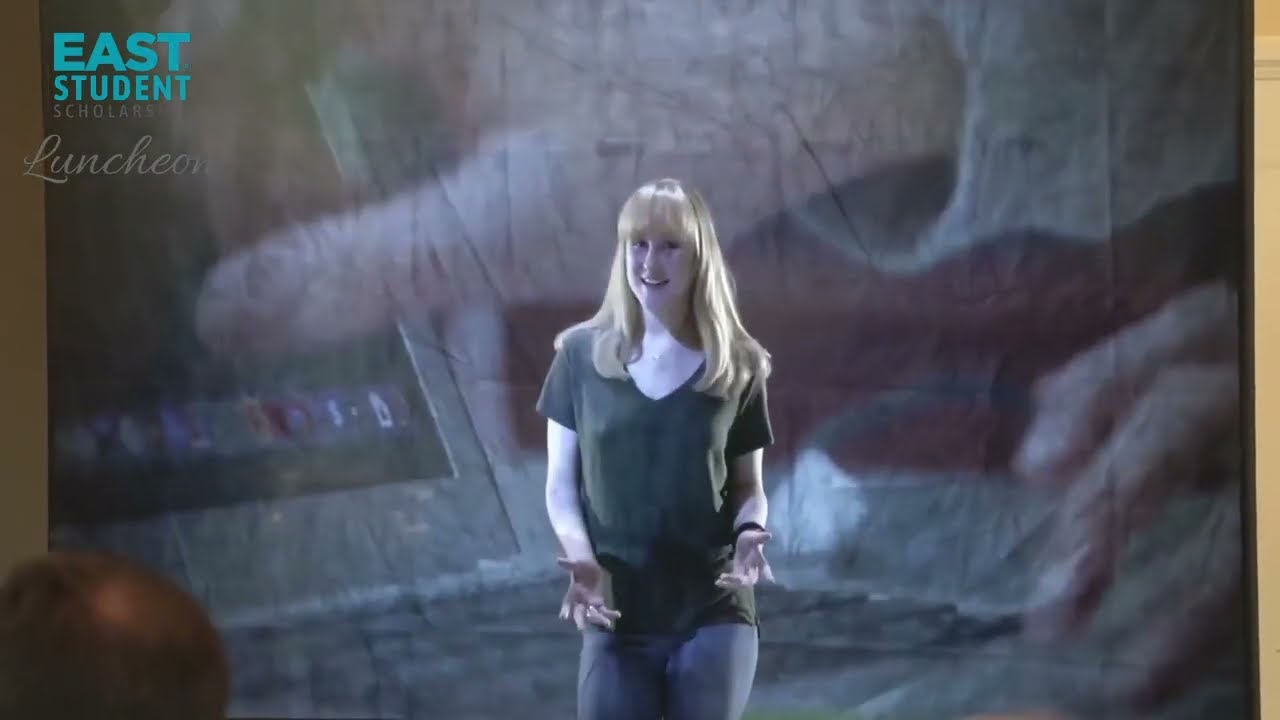In the image, there is a detailed depiction of a blonde woman with long hair that cascades just past her shoulders. She is standing centered at the bottom of the image, wearing a black V-neck t-shirt and blue jeans, presenting or teaching. Her appearance is very lifelike, yet the image has an almost graphic quality, making it ambiguous whether she is real or a digital creation. The background is a faded projection that shows a close-up of a silver laptop with a black screen and icons at the bottom. There are two hands on the laptop, one pointing towards the screen and the other touching the keyboard. The setting suggests a scholarly environment, possibly a classroom or seminar. Adding to this, in the top-left corner, text reads "East Student Scholars" in light blue and gray, with the word "Luncheon" in cursive beneath it, also in gray. The background also includes a maroon-colored vegetable or fruit in the left corner, and hands in white sleeves on some red, orange, and white books. A partial view of a man with balding brown hair is visible in the lower left corner, indicating the presence of an audience. The overall scene presents an educational ambiance, likely part of a student scholars' luncheon or presentation.